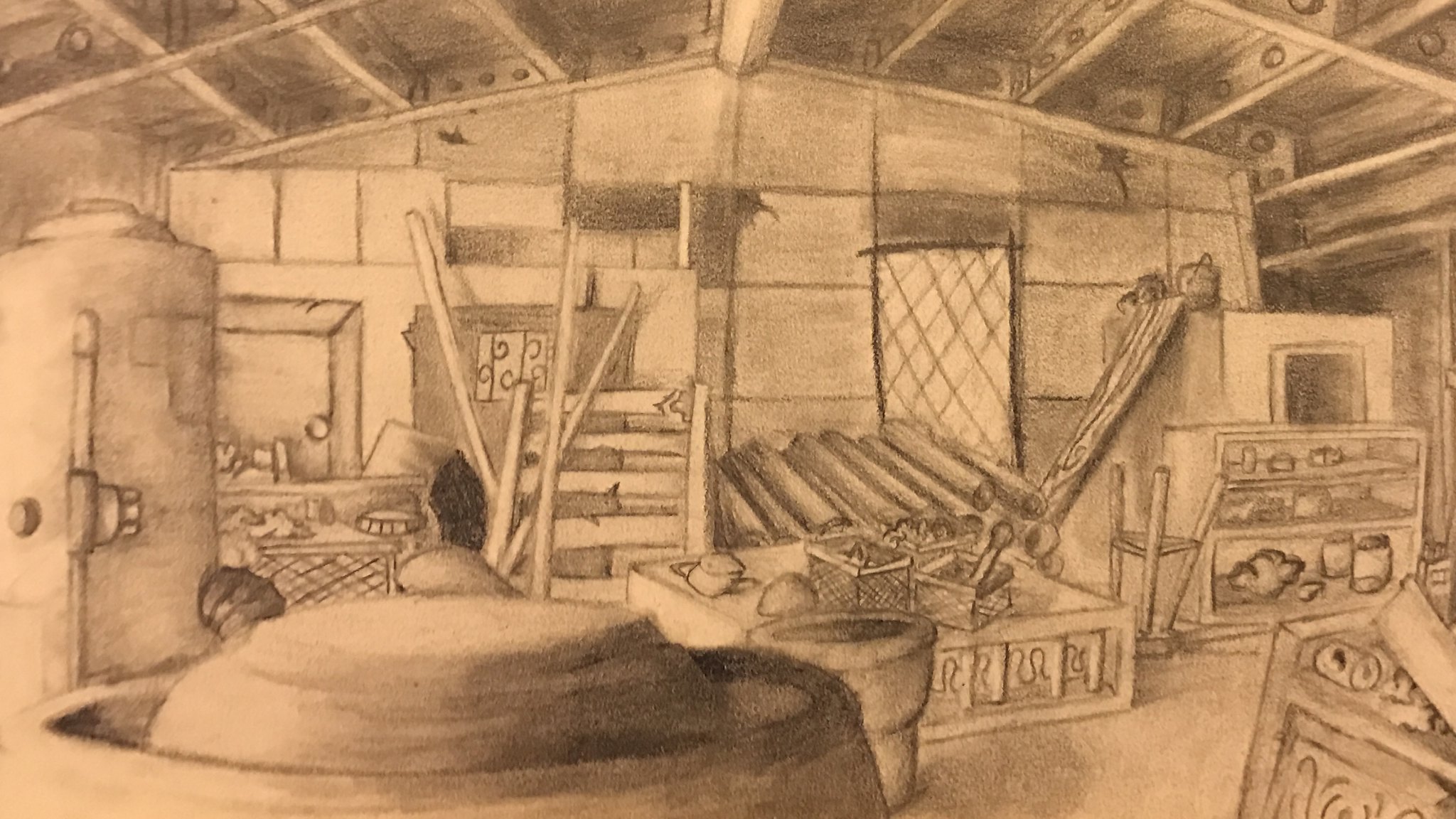This detailed, hand-drawn sketch, masterfully done in pencil, depicts a cluttered and possibly abandoned attic-like room with a vaulted or arched ceiling supported by beams. The drawing captures an array of miscellaneous items scattered throughout the space, creating a sense of disarray and storied neglect. Prominently, a sizable boiler or water heater stands almost reaching the ceiling. There are shelves crammed with knick-knacks, including jars, containers, and scrap boxes. An upside-down three-legged stool adds to the haphazard feel, while wooden pallets and pipes lie strewn across the floor. Firewood logs and tree branches are piled up, suggesting the room might have once been used for storage or practical purposes. Additionally, there are pieces of furniture, cabinets, and an enormous pot possibly for plants. The room's walls are pentagon-shaped, contributing to the unique structural ambiance, and a window offers a glimpse of light. The entire scene is shaded in grayscale, enhancing the sketch's artistic depth and intricacy.